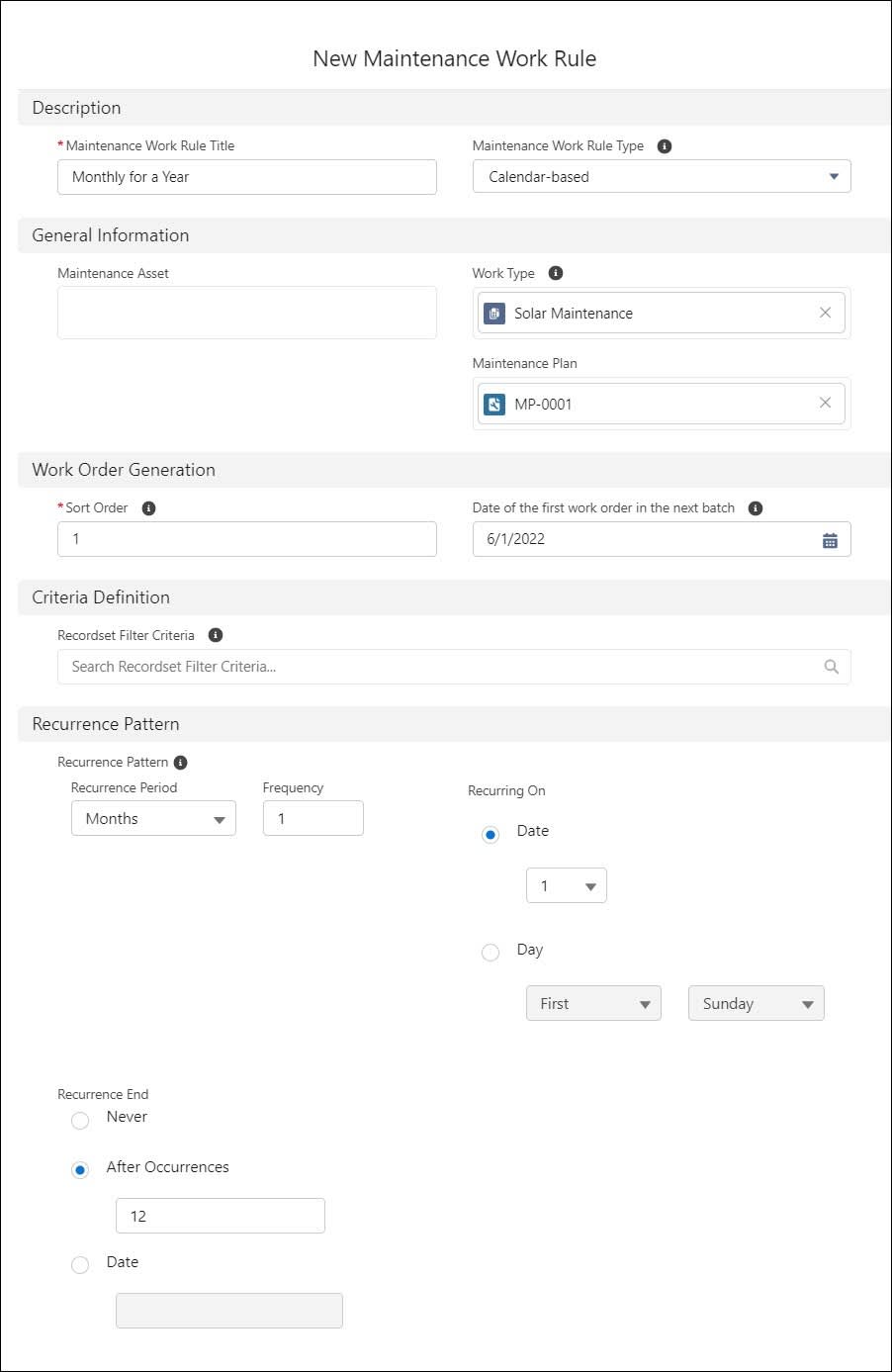**Detailed Caption of the New Maintenance Work Rule Web Page**

The web page designed for implementing a new maintenance work rule is predominantly white and structured with numerous text boxes and shaded areas. At the very top, it clearly states "New Maintenance Work Rule."

Below this header is a darker-shaded area labeled "Description." Adjacent to this section is an emphasized, weighted asterisk indicating an important note. To the right of the "Maintenance Work Rule" title, there are numerous boxes arranged in a tabular form, representing months spread across a year.

Further right is the section labeled "Maintenance Work Rule Type," accompanied by an information icon indicating it's "Calendar-Based." Below this label are lightly shaded text boxes designed for general information. 

Under the general information header, there is a box for "Maintenance Asset." To the right of this box is another labeled "Work Type," with an information icon next to it. Within this box, the term "Solar Maintenance" is mentioned, and a close-out cross is visible.

Further down the page is the "Maintenance Plan" section. Within this section, there is a box containing logos aligned to the left. Although indistinct, the logos are clearly enclosed within squares. 

The maintenance plan section also includes a case identifier labeled "MP-0001" with an adjacent close-out cross.

Below this, another shaded area is titled "Work Order Generation," including a red asterisk. The area contains fields such as "Sort Order,” also supported by an information icon and a box sporting the number "1." 

To the right is the field for "Date of the First Work Order in the Next Batch," complete with an information icon. Its associated text box is filled with the date "6/1/22," and a calendar icon is to the right.

Another shaded area titled "Criteria Definition" follows. This section features “Record Filter Criteria,” with an accompanying information icon and a search box below it that says "Search Recorded Filter Criteria."

Next, there’s a section for "Recurrence Pattern" below which lies an information icon. Fields for "Recurrence Period" are visible, containing two boxes: one for the month with a drop-down arrow and another for frequency.

Adjacent to these fields is a "Recurring On" section, where a checked bubble for "Date" is followed by a drop-down box with the number "1."

Additionally, options for specifying "Day" include two drop-down boxes for "First" and "Sunday."

At the bottom, there are recurrence settings. An unchecked button is labeled "Never," while an option for "After Occurrences" is checked with the number "12" filled in the box below it. Finally, there is another bubble for "Date" with an empty box beneath it.